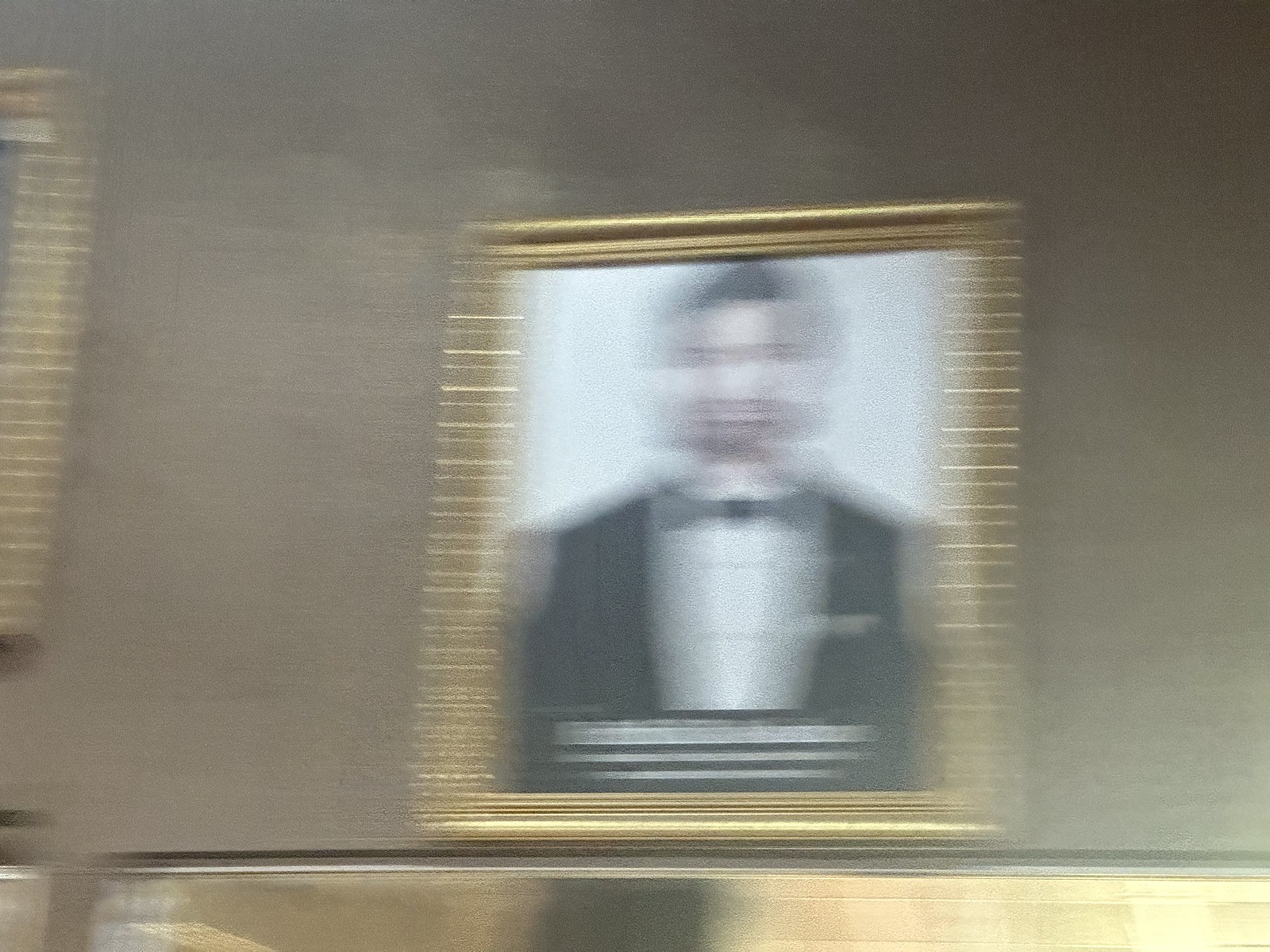A collection of artwork is displayed on a brownish taupe wall, though the image is extremely blurry. On the left side, a golden frame can be partially seen, hinting at a potentially important piece. Below, there are two other paintings, their black frames only partially visible. Dominating the center is a framed portrait that, despite the blurriness, suggests the likeness of Abraham Lincoln. The figure features a black jacket with some indistinct white text beneath it, adding to the ambiguity of the scene.